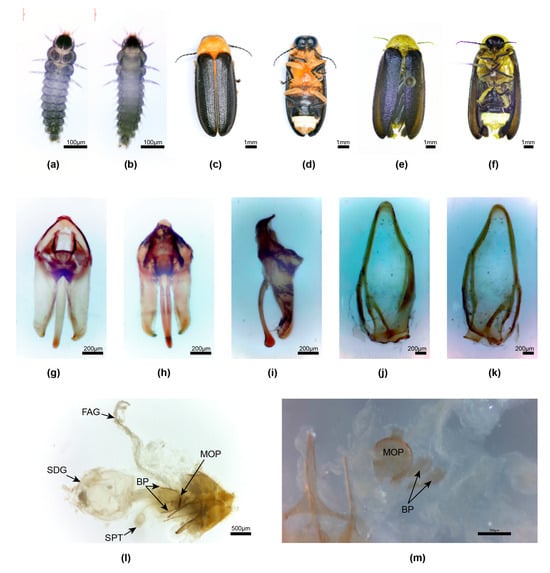The image displays a collection of specimens, potentially amoebas or small insects, arranged in three rows and labeled from A to M. The first row contains six specimens (A to F), the second row contains five specimens (G to K), and the third row contains two specimens (L and M). Each specimen is shown from different angles, with pairs such as C and D, and E and F representing the same creature viewed from the front and the back. Detailed annotations at the bottom of the image indicate specific parts of the specimens, using labels like FAC, STG, BP, SPT, and MOP. The size of each specimen is provided, giving a clear reference for scale, with measurements like one millimeter mentioned. The specimens exhibit colors primarily in browns, oranges, and yellows, with some blue hues suggesting that the image might be captured through a microscope. The overall scientific context appears to emphasize the biology of these small creatures, possibly highlighting their anatomical features and sizes.